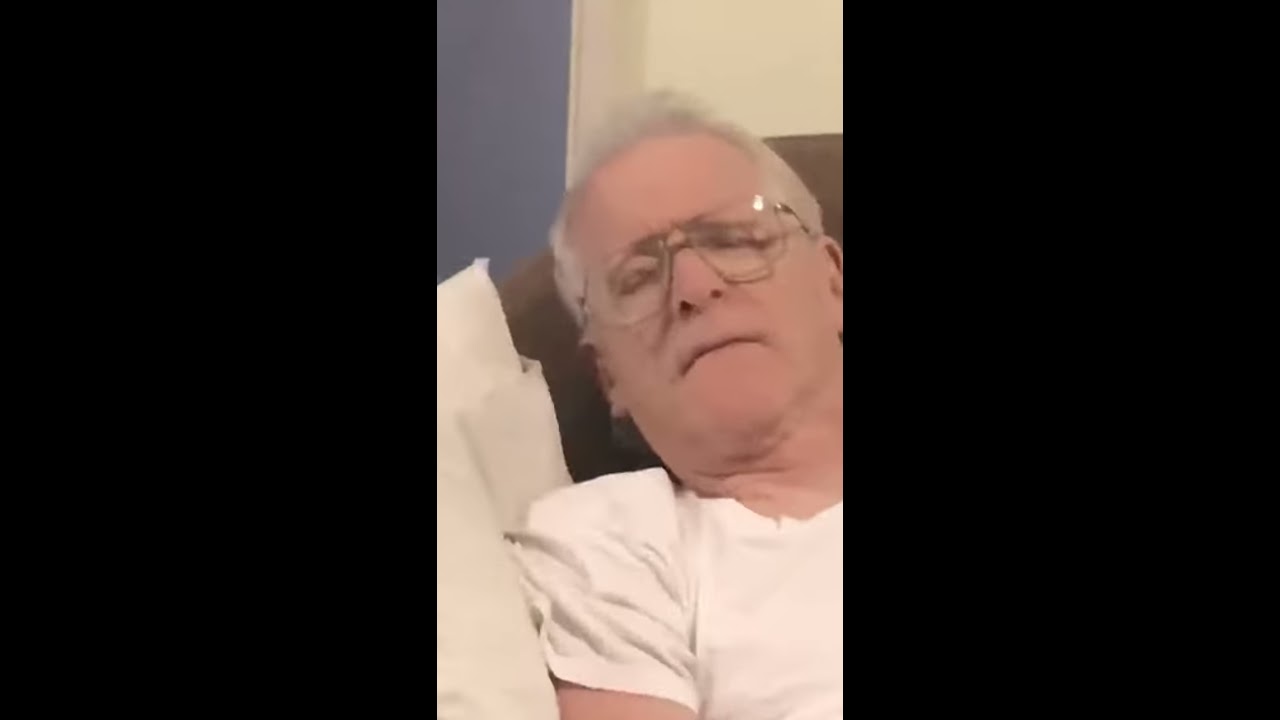The photograph features an older white man with short white hair reclining on a brown sofa, resting his head on or near white pillows. He appears to be sleeping or relaxing, with his eyes closed and his mouth turned slightly downwards. The man is clean-shaven and wears thin-framed, possibly gold glasses, which catch some light highlighting the upper right portion of his lenses. He is dressed in a short-sleeved white t-shirt. The background of the image shows a light cream-colored wall with a section of dusty blue in the top left corner, indicating the photo was taken indoors, possibly in a living room. The lighting in the room is bright, causing the man to squint slightly. Despite some wrinkles on his neck, he appears to be relatively fit and around his early 60s.